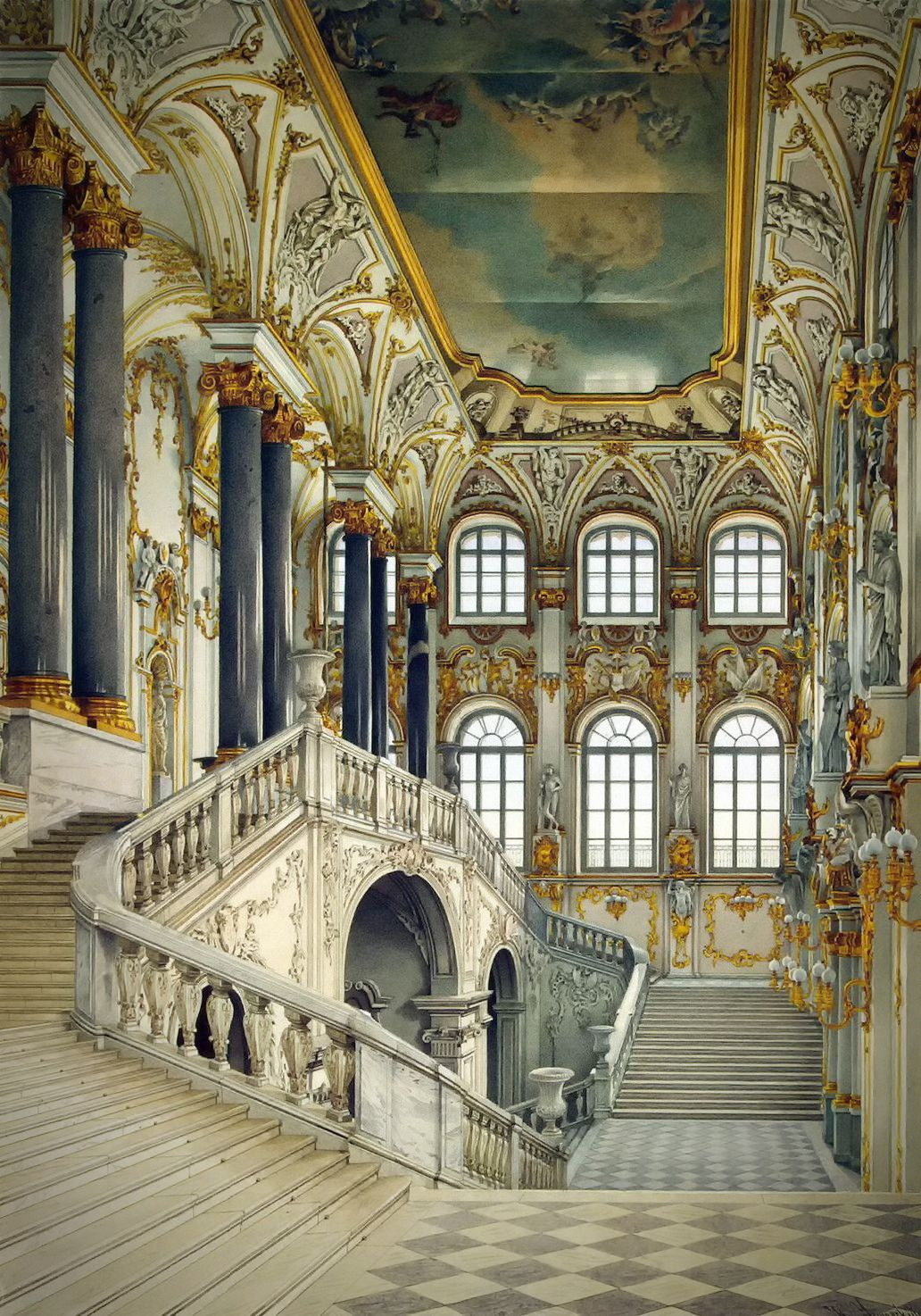The image depicts an opulent interior of what appears to be a grand palace or museum. The focal point is a grand staircase that splits into two directions, ascending to the second story, with elaborate banisters. The entire space exudes luxury, adorned in predominantly white marble with intricate gold embellishments. The ceiling features a magnificent painting rendered in whites, blues, and golds, portraying clouds, angels, and other celestial figures. The room is framed by multiple columns; the ones on the left are gray with gold capitals, while others are a darker color, lined with similar gold details. The windows have unique shapes, oval at the top and rectangular at the bottom, with the top row being smaller. The flooring consists of a striking black and white checkerboard pattern. The space is further lavishly decorated with ornate archways around the windows and finely detailed designs on the walls, emphasizing the grandiose and sophisticated atmosphere of this palace-like interior.